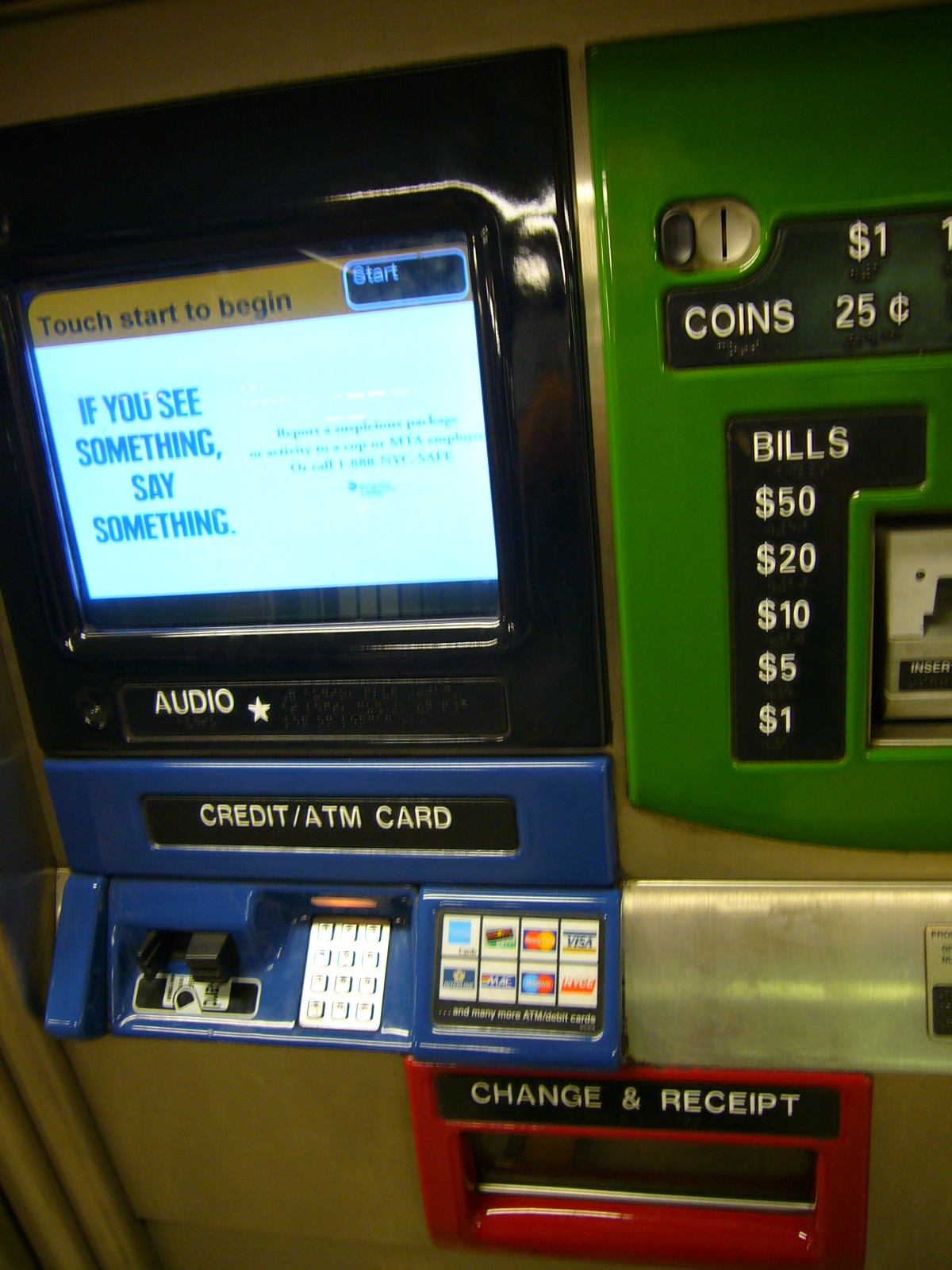The image depicts an ATM machine, focusing on the left side of the screen, which prominently displays a glowing message in large black letters stating, "If you see something, say something." Above this message is a horizontal yellow banner with black text that reads, "Touch start to begin." On the bottom section of the machine, there's a blue metal area labeled "audio," followed by "credit/ATM card." To the right, there's a red metal section labeled "change and receipt." Additionally, the top right part of the image features a partially visible panel with green metal, indicating coin and bill denominations. This section lists "coins $1.25" and "bills" in descending order from $50 to $1, with the denominations in white text and the corresponding dollar signs on the left side. The ATM machine's multiple colored sections are set against a dull yellow background.